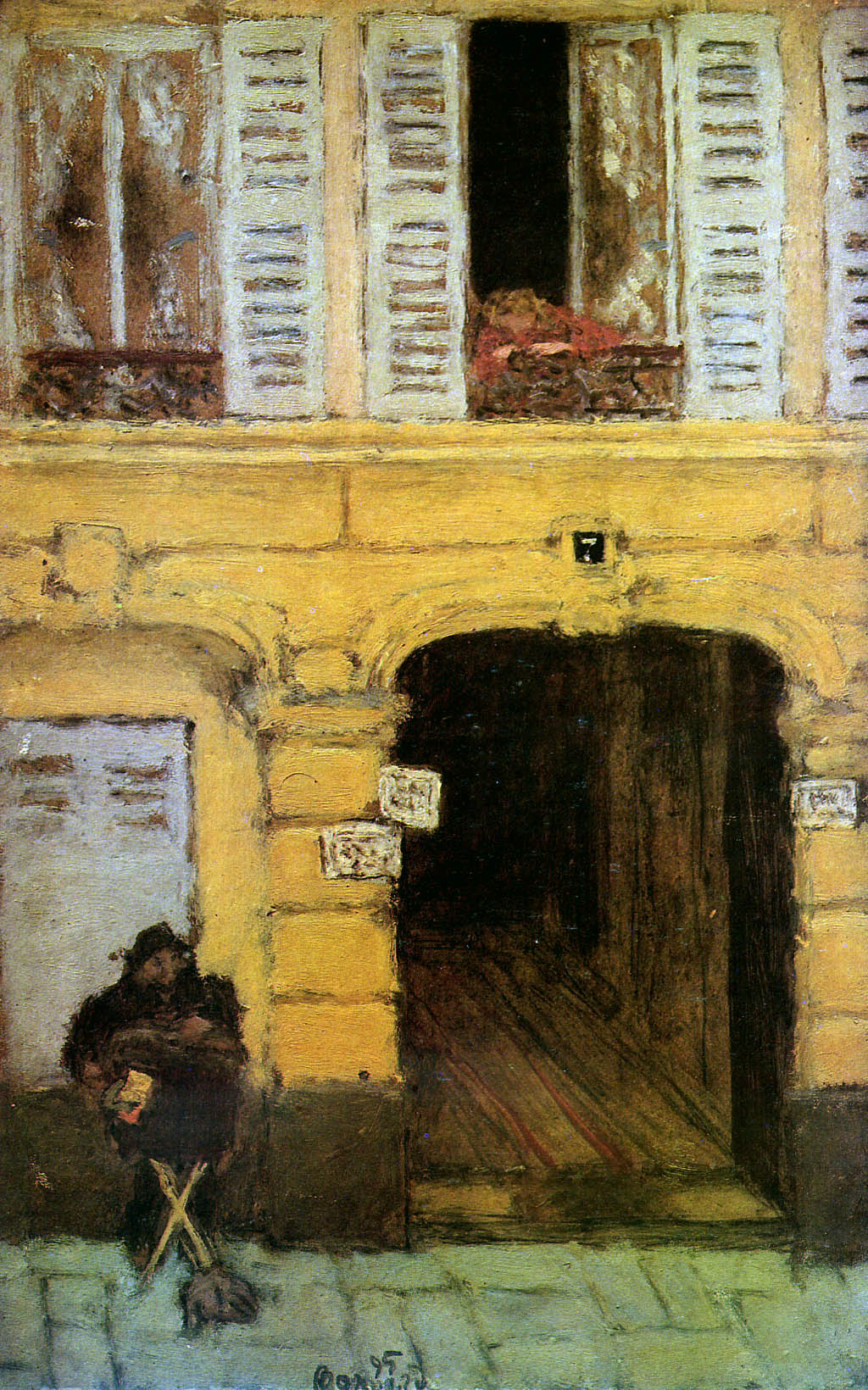This image is a detailed oil painting of a quaint town scene, evocative of historical Italian or Roman architecture. The composition is vertically long, showcasing a two-story building constructed with golden-hued stone blocks, accentuated by a cobblestone street. The ground floor features an arched entryway with a wooden floor, leading into the building. On the street, a gentleman, dressed in a hat and coat, stands holding a large black box that could be a musical instrument on a stand. The ground around him is a green-gray, resembling a brick or patio stone surface. Surrounding this main entrance are several white signs.

Above on the second floor, the building's façade transitions to a cream color, adorned with windows framed by off-white or slightly greenish shutters. One of these shutters is open, revealing a woman in an orange dress, her flowing hair adding a touch of dynamic movement. She leans gracefully over a rail, gazing out into the scene below. This picturesque setting captures the essence of a bygone era, reflecting an idyllic countryside ambiance.